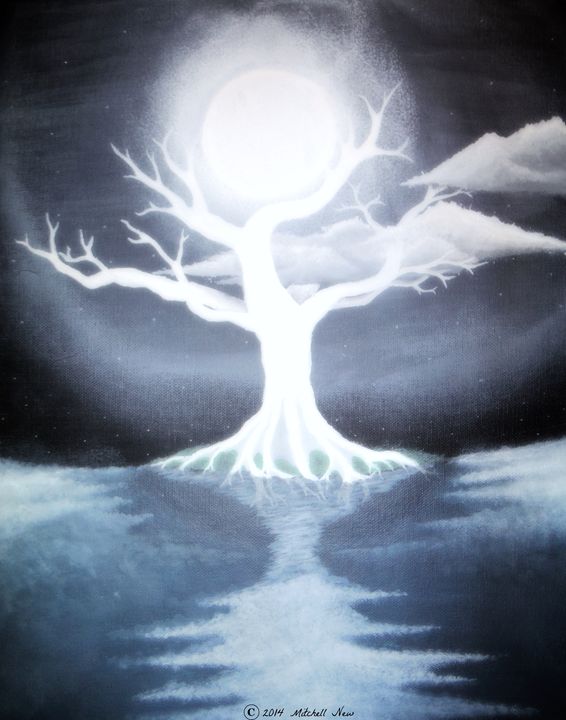This image depicts a detailed and ethereal night scene illustration dated 2014, possibly by an artist named Mitchell New, although the signature is small and written in cursive, making it somewhat difficult to read. The artwork is mainly rendered in shades of blue, black, and white, creating a dramatic and slightly eerie atmosphere. Dominating the center of the image is a luminous, leafless white tree with glowing roots that extend visibly below the ground, which may appear transparent or water-like, suggesting the tree might be growing in the middle of a lake. The tree's distinct branches arch upwards, framing a bright, full moon that illuminates the scene. Surrounding the moon are a few white clouds and tiny white dots resembling stars. The interplay of light and shadow, especially the glowing effect of both the moon and the tree, enhances the surreal and mystical quality of the artwork.